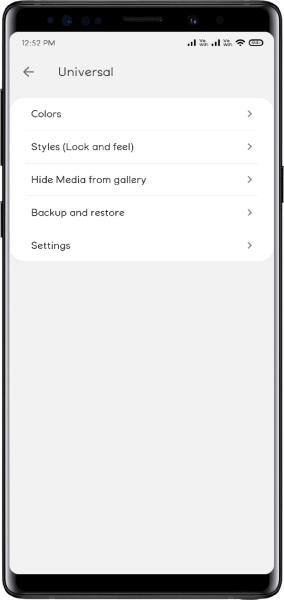The image showcases a smartphone screen displaying an app interface. The app is open, with a gray background and several main options prominently featured on white backgrounds. The text on the app is written in black, ensuring clear readability. At the top-left corner of the interface, the word "Universal" is displayed alongside a back button, represented by a left-pointing arrow.

Below the "Universal" heading, five options are listed vertically. Each option has a right-pointing arrow, indicating that more details can be revealed upon clicking. The first option is "Colours," allowing users to select a preferred color scheme for the app. The second option is "Styles (looks and feel)," which lets users customize the app's design according to their tastes. The third option, "Hide media from gallery," enables users to conceal media so that it is only accessible within the app, and not visible in the general gallery. The fourth option, "Backup and Restore," provides functionality for users to back up their data or restore it if necessary. The final option, "Settings," leads to additional settings where users can further personalize their app experience.

Each of these options facilitates a unique aspect of user customization and functionality within the app, enhancing both utility and personalization.